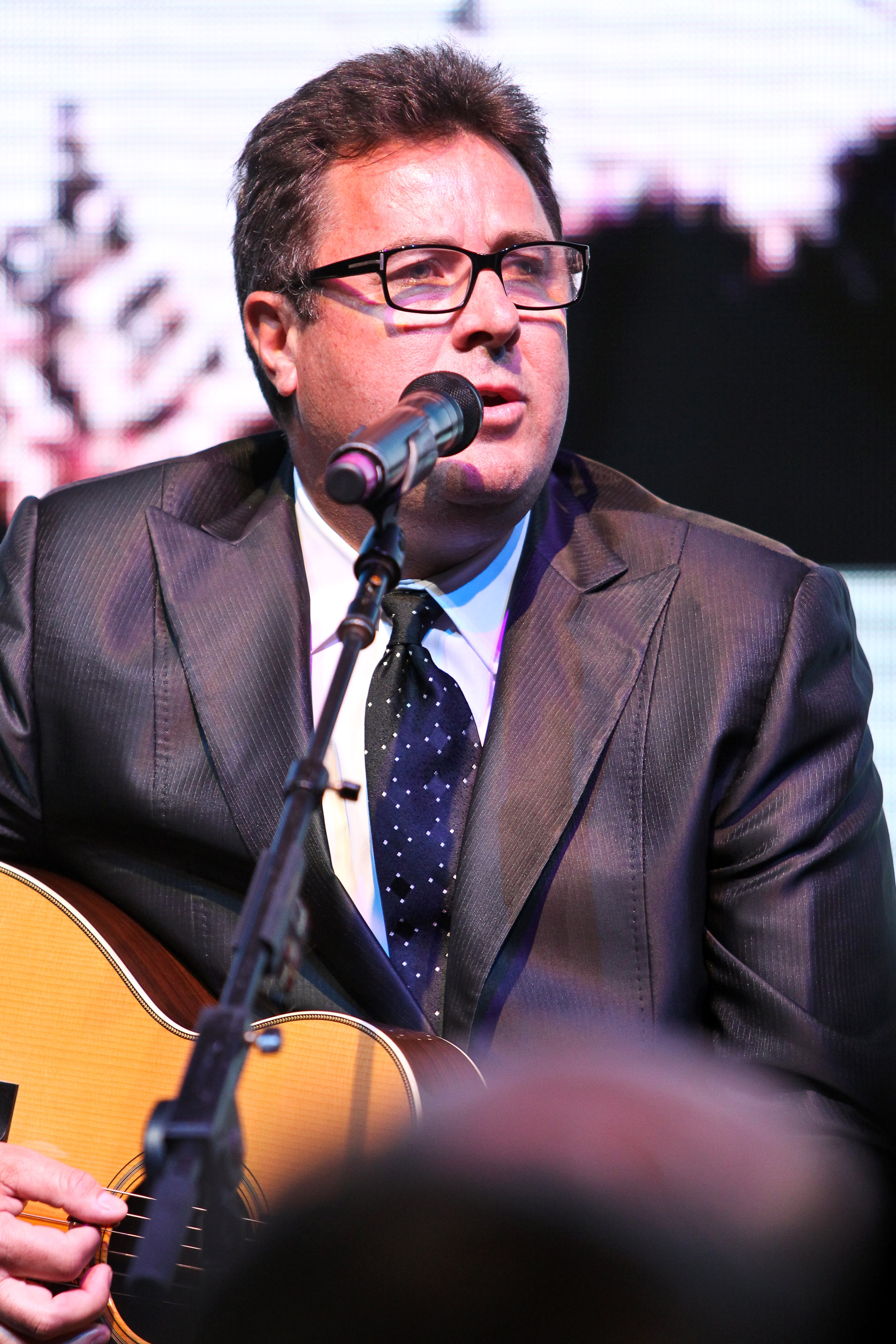This horizontally oriented, slightly squished photograph features a man who appears to be in his late 40s, of indeterminate ethnicity. He has neatly trimmed dark hair with some grey at the sides, combed back with a slightly spiky top. His clean-cut look is highlighted by somewhat rectangular black plastic eyeglasses. The man is dressed in a sharp, dark-colored suit jacket, possibly leather or a dark fabric like blue or grey. Under the jacket, he wears a crisp white button-down shirt and a dark blue tie adorned with an organized pattern of small white dots. 

The man stands near a black microphone on a stand, positioned close to his mouth, suggesting he is singing. He holds an acoustic guitar with a yellowish-tan front and a brown side, featuring a circle around its soundhole. His right hand is seen near the guitar strings, indicating he is playing the instrument. 

The background of the image is somewhat blurry, with a possible sculpture visible in the top left corner. This sculpture appears triangular with branching elements that maybe include a fish, and is surrounded by horizontal blue and white lines fading towards the bottom. On the right side, there is a dark silhouette of a line of trees. The overall impression of the image, possibly taken in the late 70s or early 80s based on its quality, blends the man's focused performance with a blend of blurred and distinct background elements, creating a nostalgic yet timeless scene.